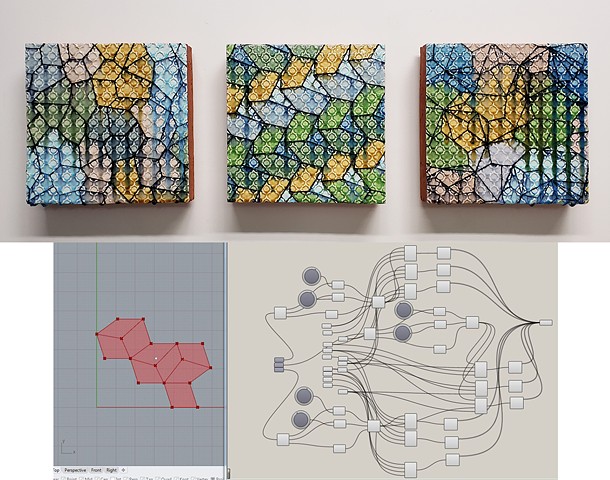The image showcases a highly detailed and unique collection of artwork, divided into three distinct sections. The top section features three square canvases, each adorned with geometric patterns in a rich palette of colors including gold, green, various shades of blue, and hints of pink. These paintings, with their mosaic-like appearance, stand out against a brownish backdrop and appear somewhat glittery.

Below the paintings, on the lower left, there is a 3D drawing resembling a cube you might see in architectural sketches. This cube is rendered in light red with darker dots and includes some unreadable text beneath it.

The piece on the lower right is a complex gray illustration that appears to be either a schematic or a network diagram. It consists of numerous gray circles, squares, and lines interconnecting various components, reminiscent of a detailed wiring diagram with little white boxes and gray colored buttons indicating different sections of the layout.